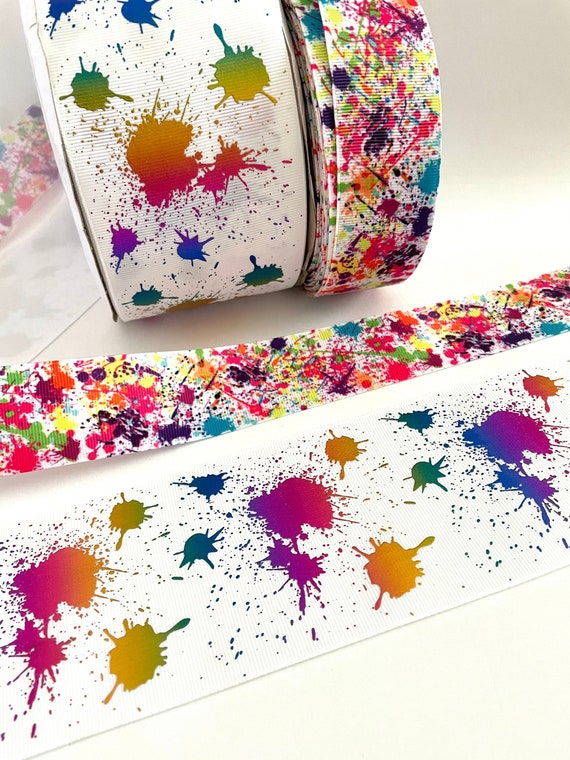The image showcases two rolls of ribbon set against a white background and white surface. Both ribbons feature a design reminiscent of paint splotches against a white backdrop. The ribbon on the left, which is rolled up, has yellow, blue, purple, pink, and smaller green splotches, with its pattern also laid flat in front for clarity. This ribbon is wider in comparison. The ribbon on the right has a higher concentration of multicolored paint splotches, including yellow, turquoise, black, orange, and violet, and less visible white space, giving it a busier appearance. This ribbon is narrower, about an inch and a half wide. Both ribbons appear to be made of either fabric or a tough material such as paper or plastic, designed for wrapping purposes.